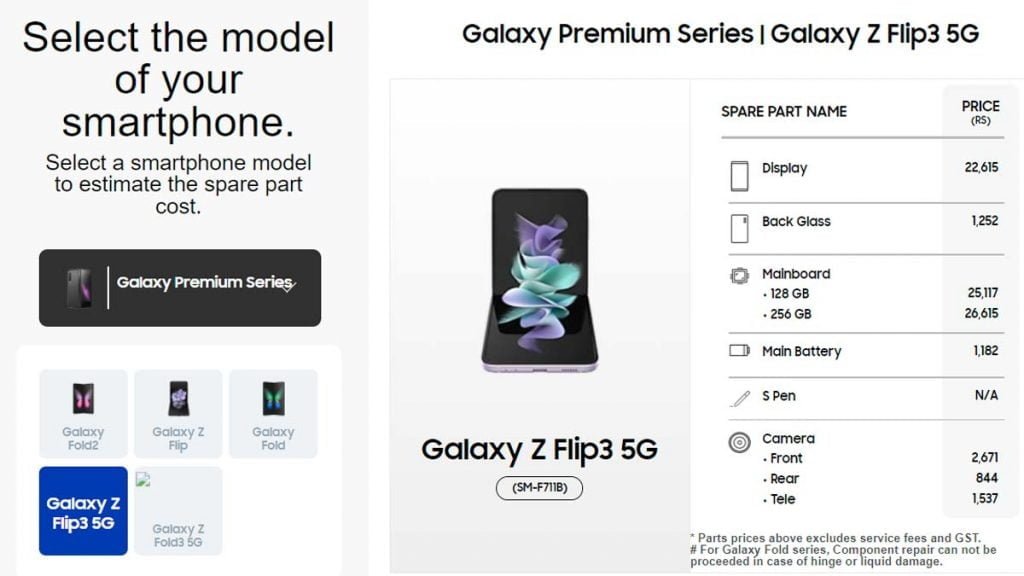A detailed screenshot shows someone attempting to purchase an Android smartphone, specifically the Galaxy Z Flip 3 5G. The pricing is displayed in a currency labeled as RS. Itemized potential costs include a display for 22,615, black glass for 1,252, a 128GB main board for 25,117, or a 256GB main board for 26,615. The main battery is priced at 1,182. Notably, the S Pen is marked as not applicable in this context. Additional spare parts include a front camera for 2,671, a rear camera for 844, and a telephoto lens for 1,537.

The prominent image in the screenshot features the Galaxy Z Flip 3 5G, distinguishable by its unique folding design, resembling a modern flip phone but maintaining a full smartphone experience. The interface prompts the user to select their specific smartphone model for comparison purposes, with options including the Galaxy Fold 2, Galaxy Z Flip, Galaxy Fold, Galaxy Flip 3 5G (selected), and the Galaxy Z Fold 5G. The visual elements and detailed descriptions in the screenshot make it clear that the user is meticulously comparing variants and spare part prices of foldable Android smartphones.